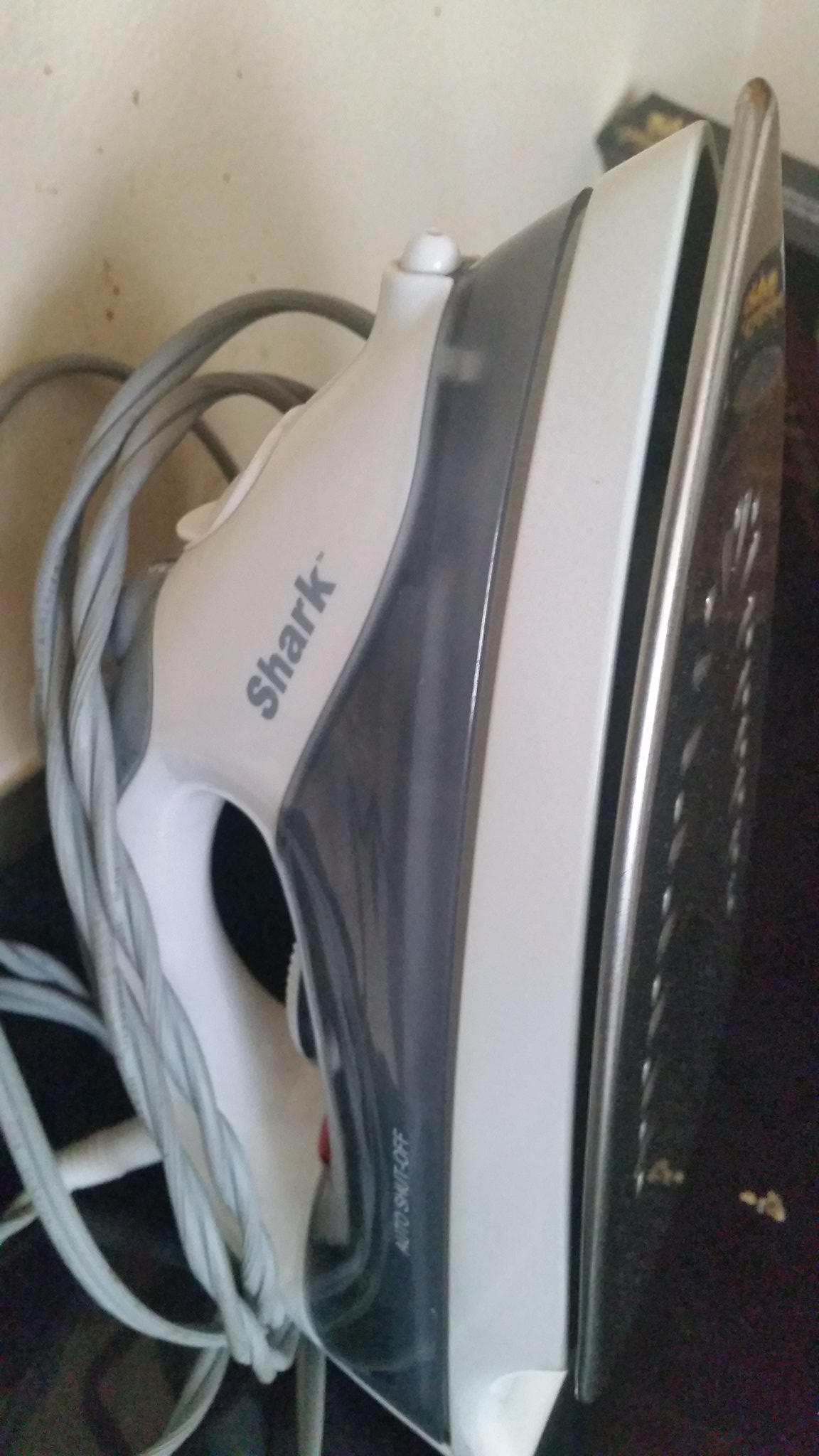This color photograph features a close-up view of a Shark brand electric steam iron, prominently displaying detailed characteristics. The iron itself is white with a central gray stripe and features a stainless steel silver faceplate, complete with holes for steam release. The brand name, Shark, is clearly written in gray letters on the white handle. A long, thin, light gray power cord is wrapped and coiled around the handle. This upright iron is positioned a few inches away from a light-colored, rather dirty wall with dark specks and shadows. Within the background of the image, partially obscured behind the iron, there is an indistinguishable black object with gold and white markings.